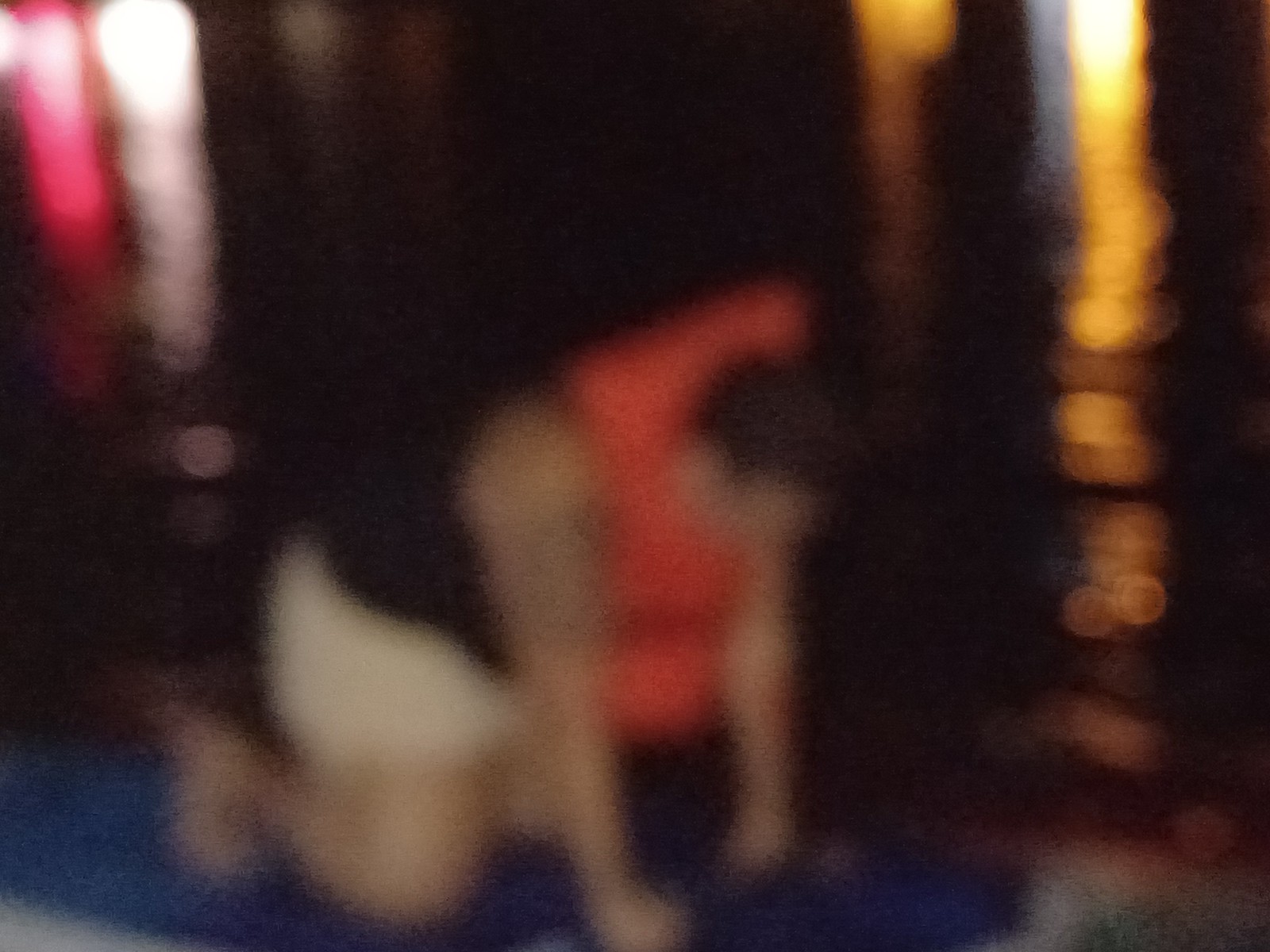A blurry photo depicts a kneeling figure with short dark hair and fair skin—presumably a man due to the short hairstyle. He is positioned on a blue yoga mat, resting on his knees with his toes touching the mat and his hands splayed out on the floor in front of him. He wears a bright orange flotation device around his neck, which extends down to his chest as he looks downward. The background consists of a series of vertical elements: a probable brown wooden door or wall, interspersed with vertical stripes of yellow-white light and dark wood on the right, and vertical stripes of white and red light on the left. The lighting variations add a striking contrast to the scene.